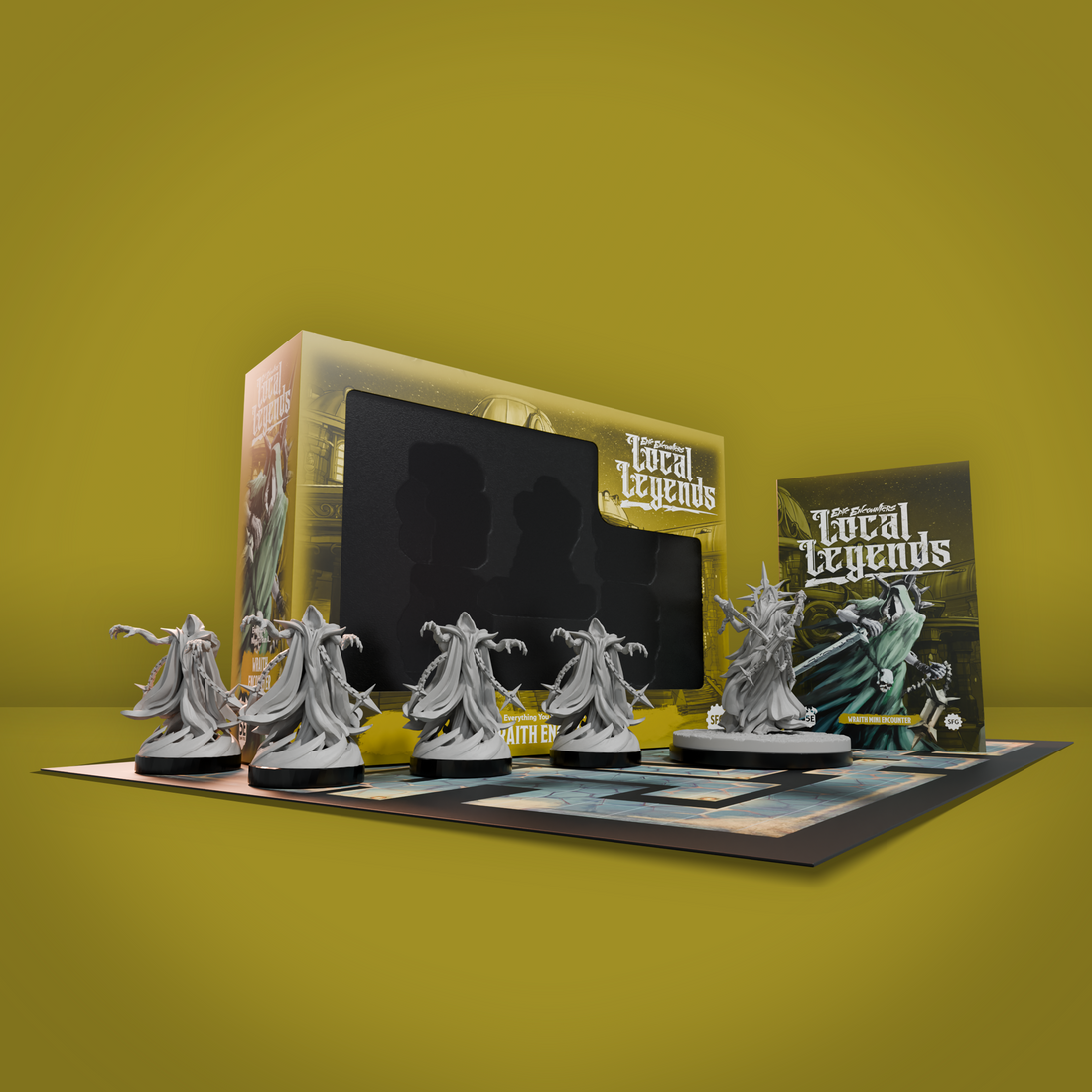The image features an advertisement for a board game called "Local Legends" set against an olive green and yellow background. At the center of the display, a blue, maze-like game board is laid out prominently, with five silver figurines positioned on top—four of which resemble ghostly figures, while the fifth appears akin to a regal King Triton character holding a sword and wearing a crown. The figurines, each with their gray bodies and black bases, are clearly distinguished. Behind the game setup, a box with a yellow design and a black center is visible, bearing the "Local Legends" title in the top right corner. Adjacent to the box, there is a booklet or pamphlet, also labeled "Local Legends," suggesting it might be the game instructions. This detailed display likely serves as a promotional image to showcase the game and its components.